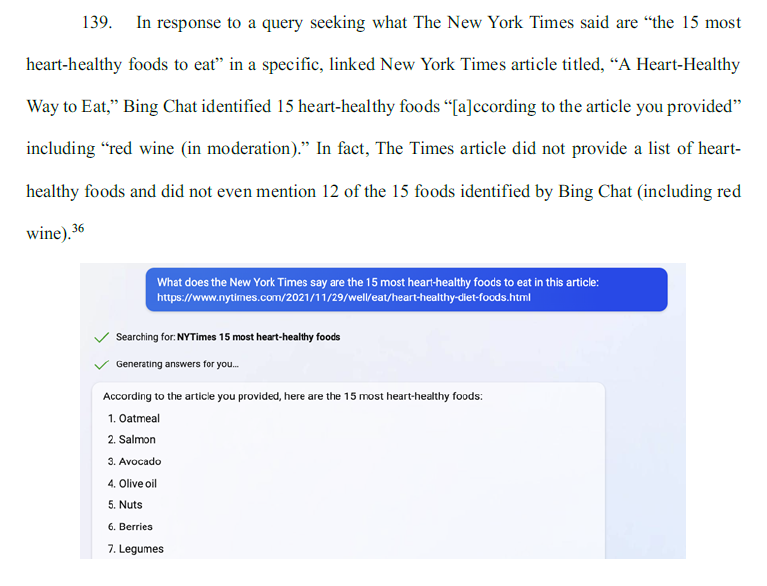**Image Caption:**

The image displays a series of messages related to identifying heart-healthy foods, as addressed by Bing Chat in response to a query referencing a specific New York Times article titled "A Heart-Healthy Way to Eat." At the top of the conversation, a message misinterprets the article, suggesting that it lists 15 heart-healthy foods, including red wine (in moderation), though the article doesn't provide such a list or mention 12 of the identified foods, including red wine.

Below this conversation snippet, a highlighted question in blue background with white text reads, "What does the New York Times say are the 15 most heart-healthy foods to eat in this article?" followed by a website link. The interface indicates an ongoing search for “New York 15 most heart-healthy food,” signified by a check mark and the phrase “generating answers for you.”

Further down, in a white square, a list purportedly from the New York Times article features the numbers one through seven aligned to the left, with corresponding food items listed on the right. These items are oatmeal, salmon, avocado, olive oil, nuts, berries, and legumes. The detailed breakdown emphasizes discrepancies between what Bing Chat identified versus the actual content of the referenced article.